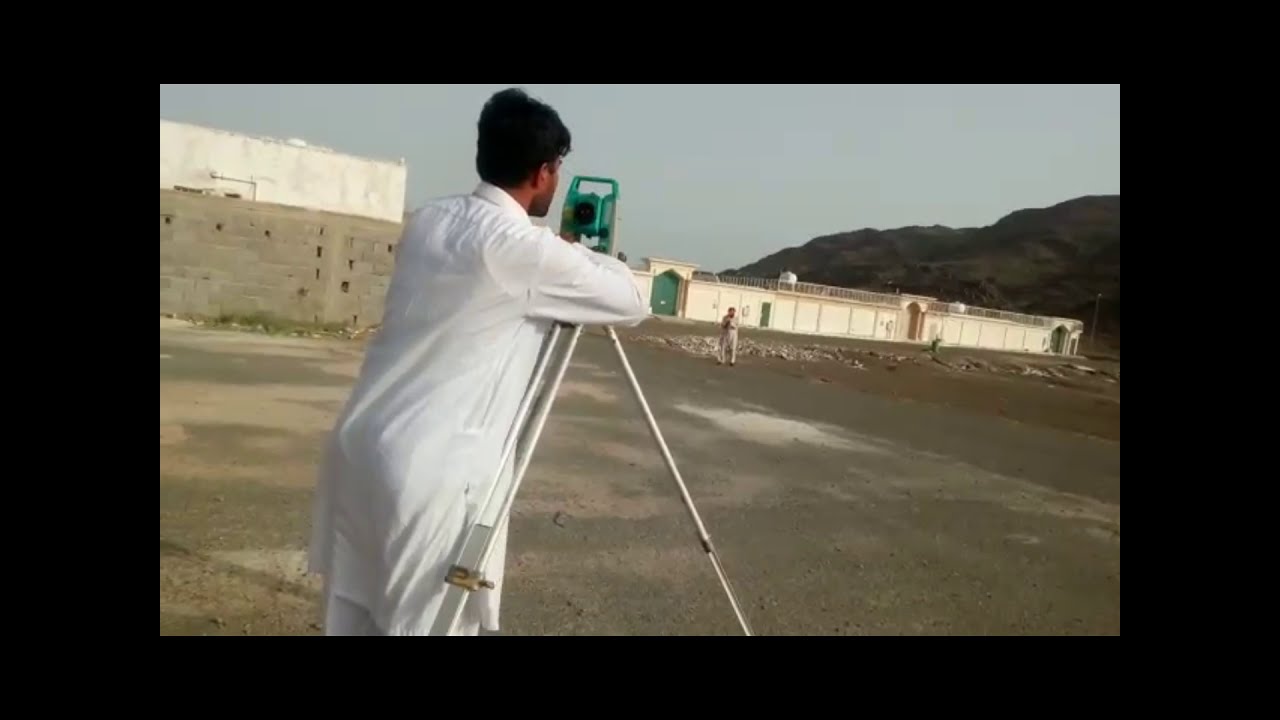The image is a horizontally rectangular photograph framed by a thick black border, with the sides being broader than the top and bottom. It captures the backside of a man, likely of Indian or Middle Eastern descent, characterized by his short black hair, darker skin, and a bit of stubble visible on the right side of his face. He is donned in a long white coat resembling a doctor's jacket or an Indian robe, and is positioned in a parking lot with what appears to be a wet ground varying in darkness.

The man is intently looking through a sizable green camera mounted on a silver-legged tripod, pointed towards a distant mountain under a blue sky in the upper right corner. To his left, there stands a high stone wall or building, brown in color, that obscures most of a white structure behind it. The setting includes elements suggesting a flat terrain with dirt and grass patches, and a large gated archway visible in the backdrop, evoking a sense of surveying land.

Additionally, there is a second man in the far background, similarly engaged in using surveying equipment and looking towards the man in the white coat. The surroundings hint at a location possibly in the Middle East or India, framed by mountains and hills on the right and various walls and buildings scattered throughout.